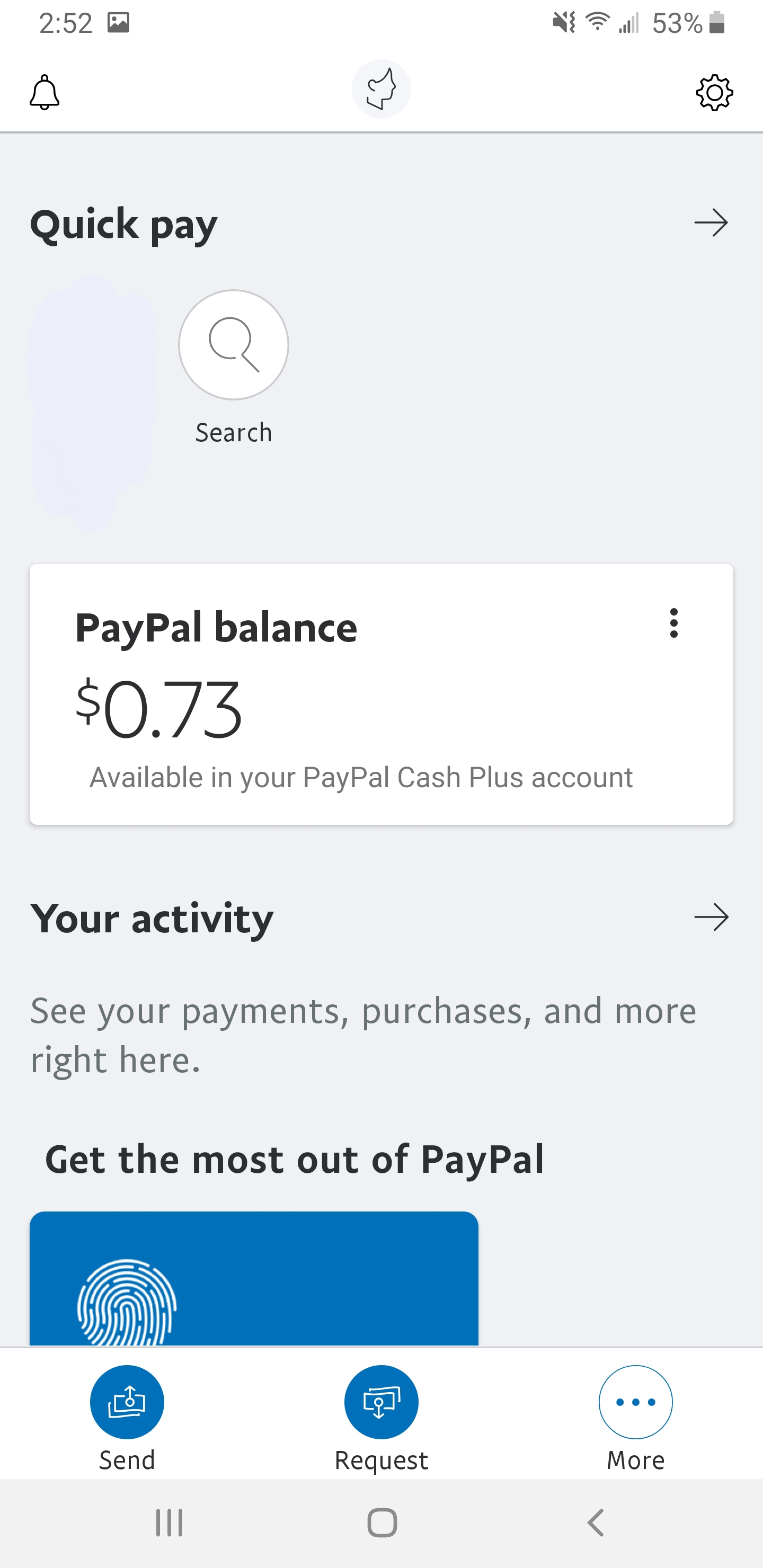The image showcases an Android phone screen, displaying the PayPal app's main interface. At the top of the screen, it is 2:52 p.m., with full WiFi connectivity, two bars of phone signal, and the ringer muted. The battery icon indicates 53% remaining battery life. 

The PayPal app interface includes a "Quick Pay" and "Search" option at the top. Below it, a rectangular box highlights the PayPal balance in black font, showing $0.73 available in the PayPal Cash Plus account. Underneath, there is a section titled "Your Activity" with an arrow for navigating to details, offering insights on payments, purchases, and more, displayed in a lighter gray font.

Further down, in black font again, it says "Get the most out of PayPal," accompanied by a blue field showing a fingerprint icon. Below this field are three buttons: the first two on the right are blue. The first button, labeled "Send," features a money symbol and an upward arrow, while the second button, "Request," displays a money symbol with a downward arrow. The third button, labeled "More," is represented by a kebab menu with three vertical dots.

At the bottom of the screen, the standard Android navigation panel is visible, consisting of three icons: three horizontal dashes on the left, a circle in the center, and an arrow pointing left on the right. The overall interface is clean, with black and blue as the primary colors, providing a straightforward user experience.